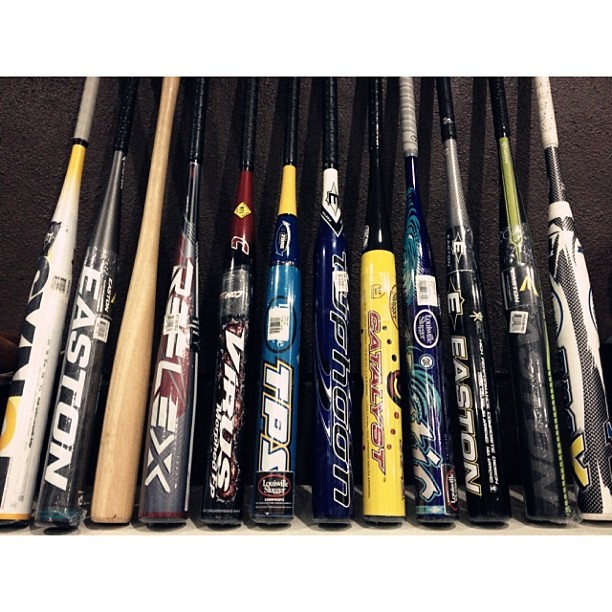In this detailed landscape-oriented photograph, twelve baseball and softball bats are meticulously lined up next to each other against a black wall, resting on a white floor. Each bat is positioned vertically, showcasing an array of distinct designs and vibrant colors. The lineup begins on the far left with a white softball bat that features black text. Adjacent to it is a black Easton bat with white text. The third bat is a wooden one with a notably skinny barrel. The fourth bat, adorned with "Reflex" in white text, flaunts a mix of red and silver hues. Next in line is a red and black bat branded with "Virus" in white text. The sixth bat stands out with its dark blue barrel embellished with yellow towards the end, branded as TPS. Following it is a dark blue Typhoon bat outlined in white. The eighth bat is a bright yellow Catalyst with red text. Next is a Louisville Slugger with white text, featuring light blue swirls against a dark blue background, resembling a fingerprint pattern. The subsequent three bats are from Easton: one black with white text, another all black with light gray text, and the last a blend of yellow and black. Each bat's unique color scheme and branding contribute to the diverse and visually striking collection.